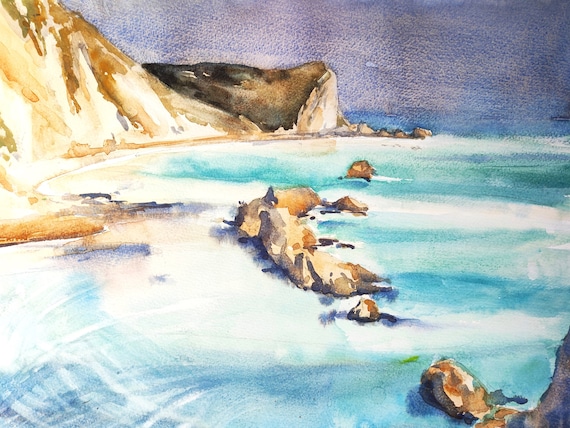This detailed painting, rich with a palette of colors ranging from purplish-white, lilac, and dark blue to various shades of brown, teal, and golden yellow, captures a serene seashore scene during the day. The moderately square canvas, without any distinct border, depicts the meeting point of land and sea. Dominating the left-hand side of the painting are two large rock formations, their hues blending light browns to dark black. These rocks stand tall, surrounding a lighter brown sandy cliff that gradually slopes towards the foaming teal blue water. Scattered throughout the shallow water and towards the center of the image, smaller rocks pierce the surface, their colors mirroring the larger formations. The upper right portion of the painting features a sky transitioning from purplish-white to dark blue, illustrating a tranquil coastal atmosphere. Brush marks can be seen throughout, adding texture and depth to the scene, capturing the movement of the foamy waves that gently lap at the shore and rocks.